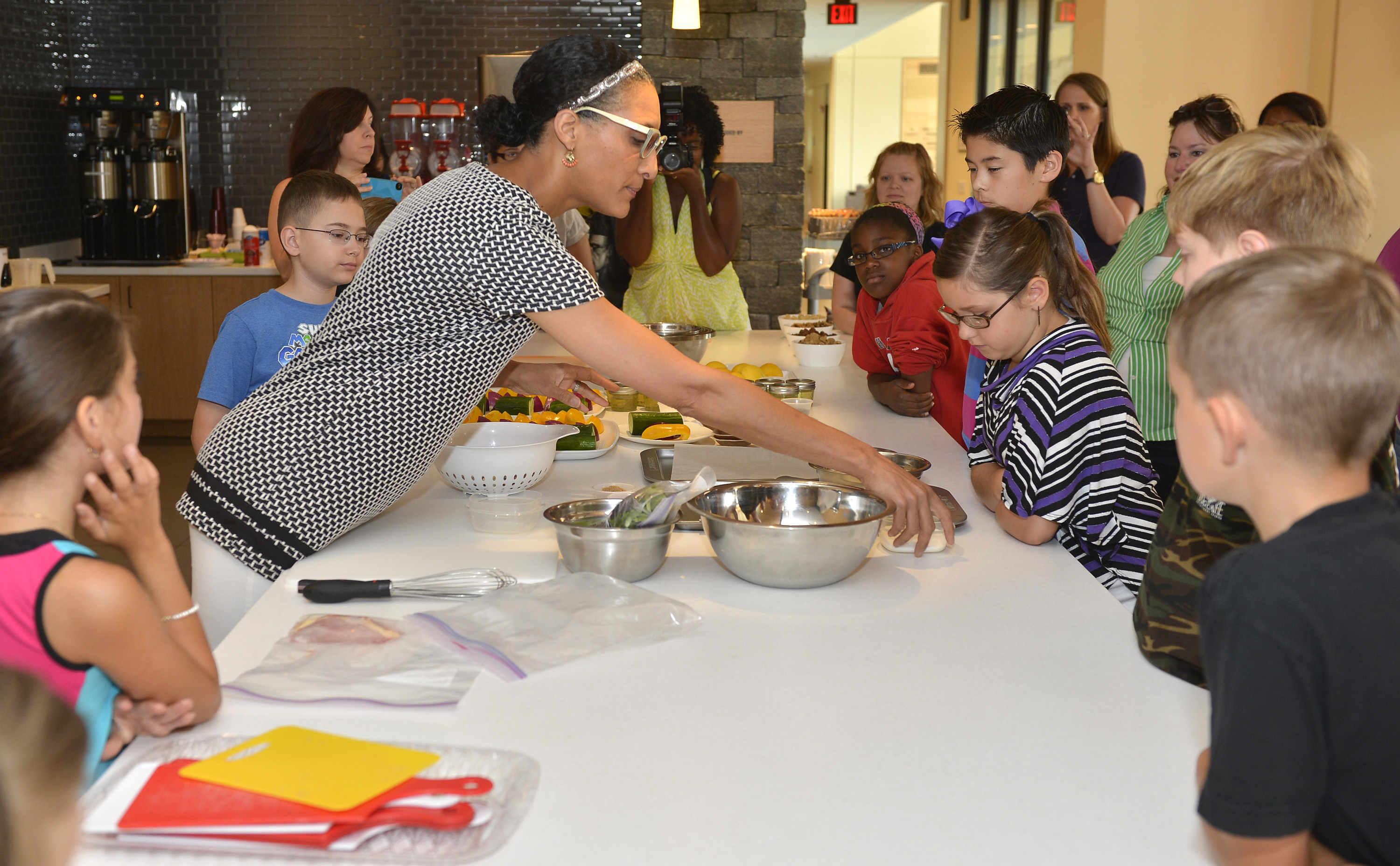The photograph captures a bustling cooking demonstration in a public building, likely a school or community center, identifiable by an exit sign and a hallway in the background. Central to the image, a middle-aged woman with short black hair, glasses, a headband, and wearing a black and white top with white pants, is actively engaging a group of at least half a dozen children gathered around a large white table. The children, some of whom are wearing glasses, are intently watching the woman as she reaches over the table, possibly preparing a meal or teaching them how to cook. The table is crowded with various cooking ingredients like lemons, metallic pots, plastic strainers, utensils, bowls, and small plastic bags. Additional background details include an adult in a yellow dress who is taking photographs of the scene, and several coffee makers. The overall setting suggests a lively and educational atmosphere where both children and adults are immersed in the cooking activity.